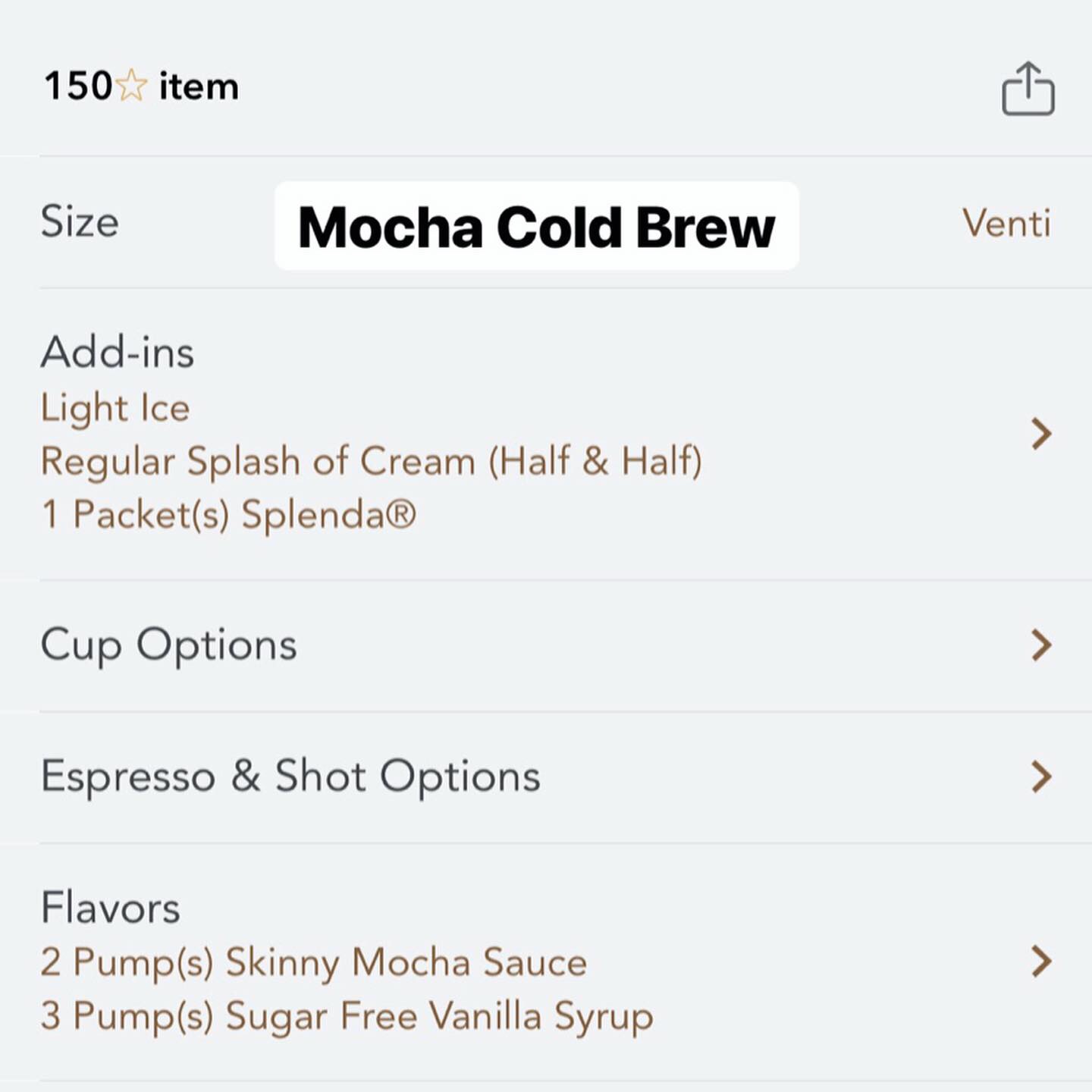A detailed and descriptive caption for the image would be:

On a light gray background, there is a rectangular screen design. In the top left-hand corner, bold black text displays the number "150" followed by an unfilled gold star and the word "item" also in bold black text. On the far right side of this top line, a download icon is present. A faint, thin gray line runs horizontally just below this top section.

Beneath this line, the word "size" appears in black text on the left side. Centered on the page in bold black text, and highlighted with a white box around it, is "mocha cold brew." To the right of this, in red text, is the word "venti." Another thin gray line is situated underneath this section.

Following this line, the word "add-ins" is presented in black text on the left side. Below "add-ins," in dark red text, the list includes "light ice," "regular splash of cream (half and half)," and "one packet (S) Splenda." A forward arrow is also displayed in this section. Another thin gray line separates this block of text from the next.

The words "cup options" in black text, followed by a forward arrow, head up the next section, which is also separated by a thin gray line from the next one.

The subsequent section is titled "espresso and shot options" in black text, delineated by yet another thin gray line.

Finally, at the bottom of the screen, the word "flavors" in black is followed by details in red text: "two pumps skinny mocha sauce" and "three pumps sugar-free vanilla syrup."